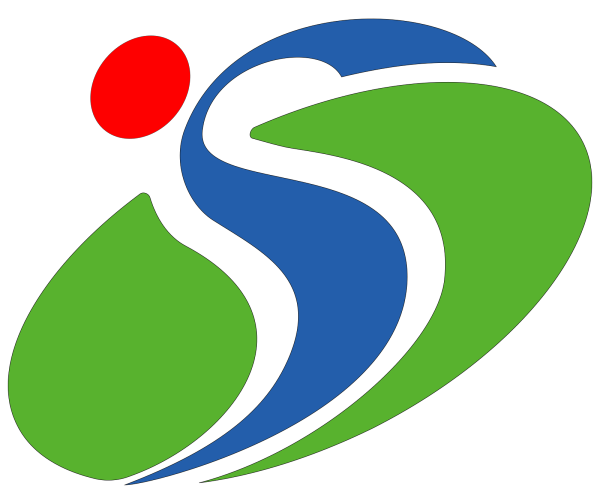The image presents a vibrant, creative logo set against a stark white background, emphasizing its design elements. Central to the logo is a prominent blue "S" shape, which starts wide at the top, narrows towards the middle, and then broadens again before tapering off to the left into a thin tail. This "S" is flanked on the left by a green, wide teardrop-like shape, and on the right by a green, backwards-curved "C" shape, both contributing to the logo's dynamic flow. A small red circle, positioned at the top left corner of the central blue "S," adds a striking accent. The overall composition, devoid of any text, suggests a modern, abstract aesthetic likely intended for company branding or digital presence.